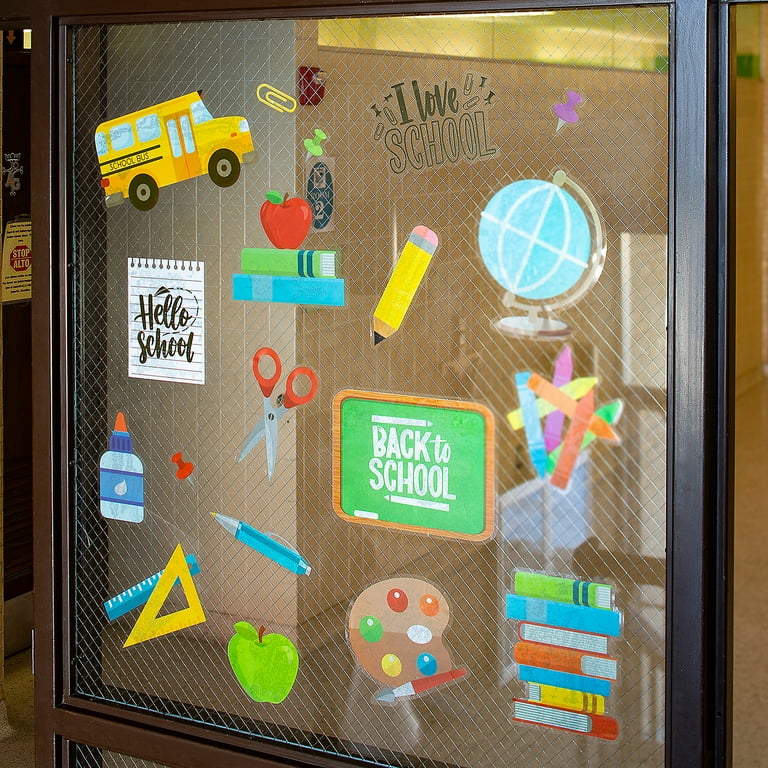In this realistic photograph, we see the top pane of a door in the interior of a school building. The glass pane, which is framed in a dark black or brown metal frame and reinforced with wire mesh, is decorated with an array of vibrant, cartoon-style stickers celebrating school. The scene captures a collage of educational-themed images, including a variety of school supplies and symbols. From the top, the stickers include school books, a paper clip with "I love school" written on it, a thumbtack, and a piece of paper that says "hello school" among other items. Further down, there are additional stickers such as a school bus, an extra-large pencil, a push pin, a globe, a cluster of crayons, a small blackboard with "back to school" written on it, scissors, glue, rulers, a paint palette, and multiple stacks of books. In the background, a hallway with beige tiles and white grout is visible, and a white piece of paper with a blue circle marked "2" can be seen, hinting at the school's layout. This detailed collage highlights the lively and welcoming school environment.